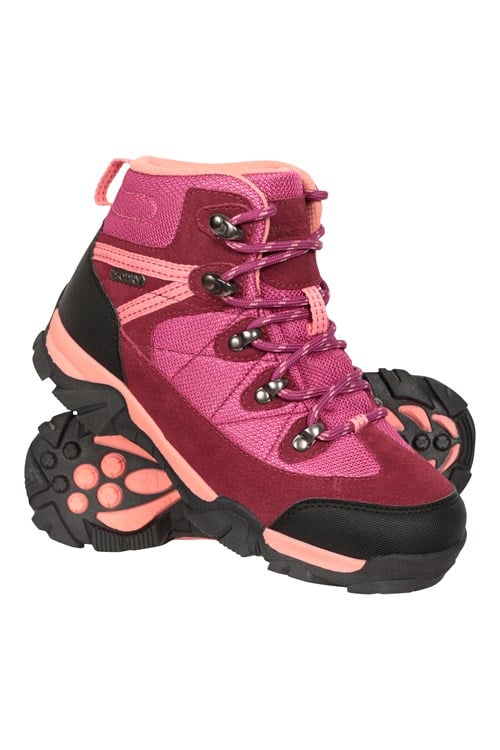This detailed color photograph features a pair of small-sized children's athletic shoes. The image is vertically oriented and uses a clean, white background that emphasizes the shoes without any external distractions. The top shoe is propped up at an angle, resting on another shoe lying flat, exposing its bottom tread. These are high-top sneakers, predominantly pink with variations in hue. The main fabric of the shoe is a lighter pink, while dark red leather trim accentuates areas around the laces, ankle, and the bottom sole. 

The ankle area features a salmon-colored trim, adding a subtle distinction in hue. The sole itself is black rubber, adorned with a salmon stripe that encircles the bottom and extends over the toe. The bottom tread, prominently displayed, is primarily black with significant light salmon detailing. Dark pink laces with lighter pink accents weave throughout the lacing system, contributing to the overall textured appearance of the shoe. The high-top design includes pink padding inside and a fabric loop at the back. The photograph adheres to a realistic, product-focused style, presenting the shoes as if floating against the white backdrop.